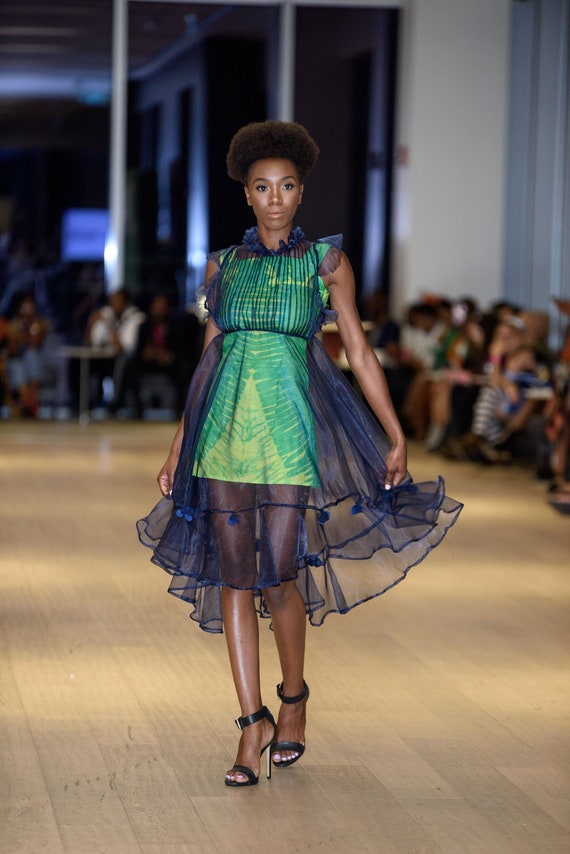This image captures a black female model striding confidently down a runway at a fashion show. She stands as the focal point in the middle of the frame, with her presence emphasized by a striking outfit and poised demeanor. Her short black afro, neatly styled and cut at the top of her ears, complements her youthful appearance, suggesting she is around 25 years old.

The model exudes elegance in a sheer blue overlay dress that offers a glimpse of the neon green mini-dress beneath, which features a design reminiscent of large banana leaves, symmetrically mirrored on each side. Her ensemble is completed with black high-heeled shoes, each adorned with a strap and a silver buckle around the ankle. 

Surrounding the runway, spectators sit attentively along the edges of the room, observing from seats situated beside large mirrors. The hardwood floor beneath the model extends backward, adding depth to the scene and anchoring the setting of this dynamic fashion show. The colors in the image are vibrant, with greens, yellows, browns, blues, pinks, tans, whites, blacks, and grays creating a vivid and lively atmosphere.